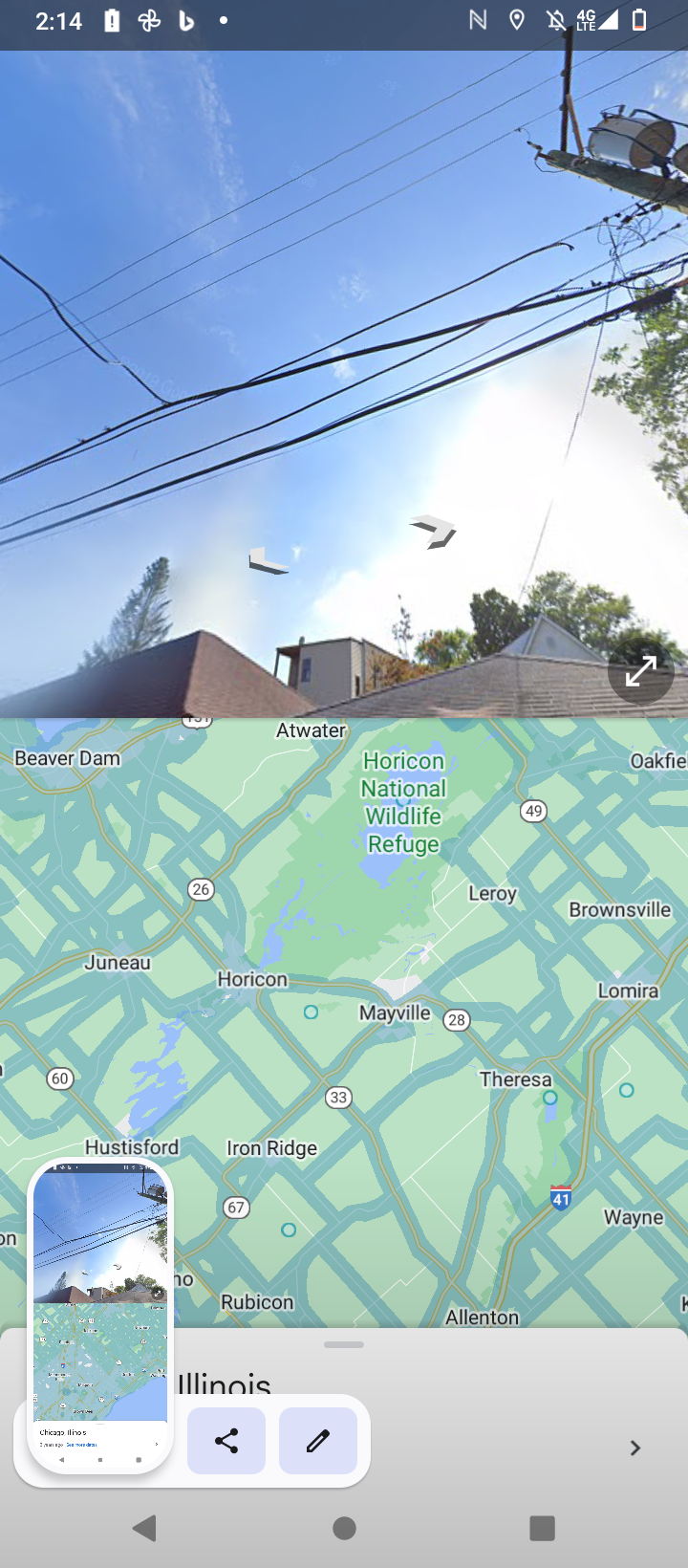This screenshot, taken from a vertically oriented smartphone using a map application, vividly captures both a street view and a map interface. The top half of the screen features a street view image depicting a bright blue sky partially obscured by a white cloud in the bottom right corner. In this section, a network of power lines stretches from the top right to the left center, crossing over the roofs of some buildings, likely houses, with their roofs cut off at the frame's bottom. Notification icons adorn the top border, indicating a low battery, 4G LTE signal, app alerts, and more.

Below the street view, the bottom half of the screen displays a map. The map is predominantly green, showing teal-green roads and a large dark green area labeled "Horicon National Wildlife Refuge." The map section seamlessly integrates a smaller, inset image of the street view, delineated by a white rectangle with rounded corners in the bottom left.

Accompanying this display, the smartphone's interface subtly reappears at the screen's bottom edge, showcasing navigation icons including arrows, a circle, and a square, against a dark gray backdrop. The layout emphasizes essential map details, such as street names and landmarks, highlighted in black text with white edging, ensuring clarity and ease of navigation.